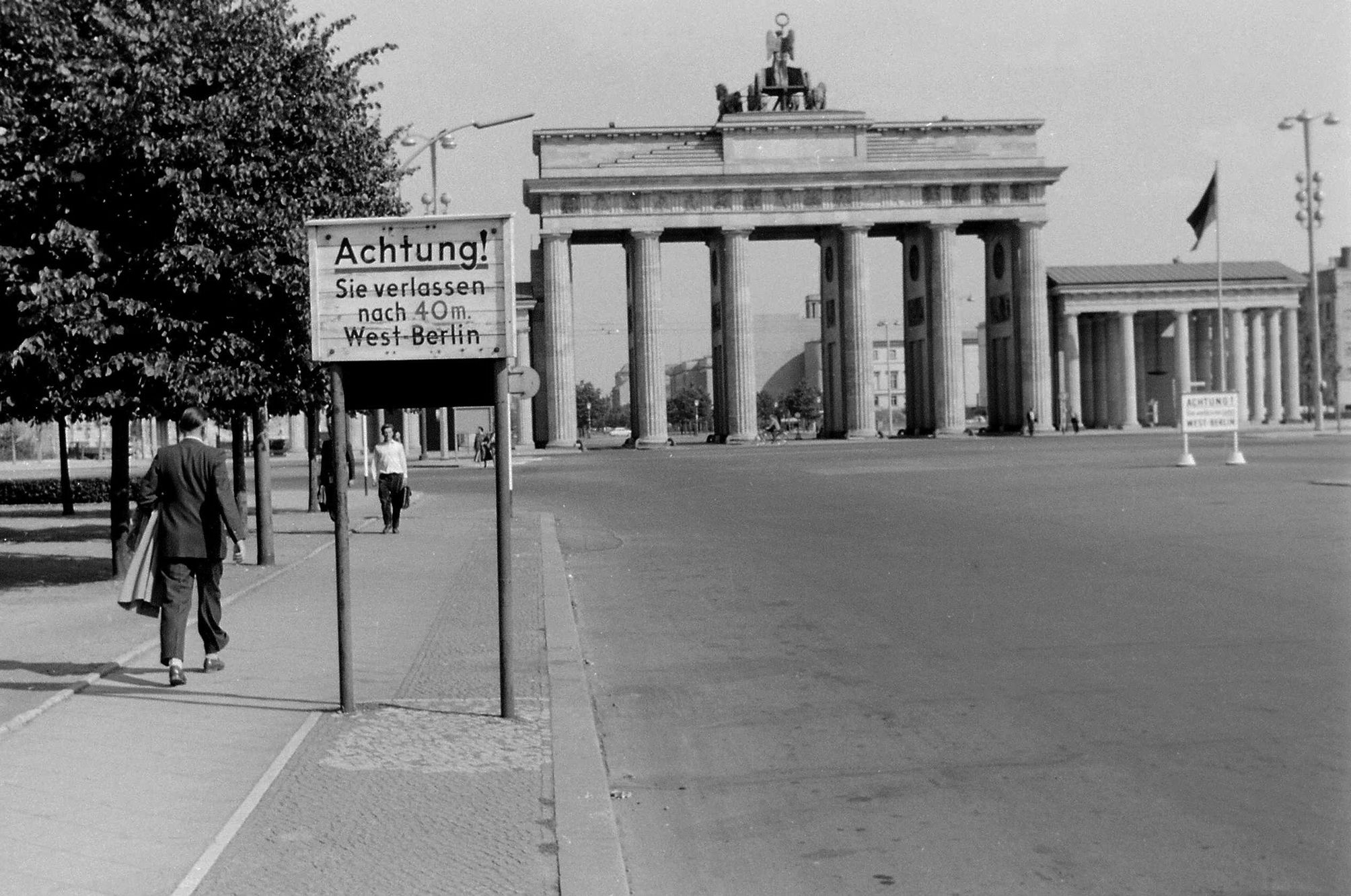This black-and-white photograph captures a moment on a bustling sidewalk, presumably in Germany, as suggested by the German sign that reads "Achtung! Sie verlassen nach 40M West Berlin." The main subject is a gentleman walking to the left, holding a coat under his left arm, and almost passing under a tree. To the right of him, the sign reinforces the German setting. Further down the sidewalk, another man in a white shirt and black pants approaches, along with a couple in the background also walking his way. Dominating the middle background is a large, ornate structure crowned with an angelic sculpture atop white pillars. To the right, a smaller version of this building with five pillars stands, accompanied by a flag in front. The absence of vehicles and modern street clutter suggests this photograph was taken a long time ago, capturing a serene yet historically rich scene.